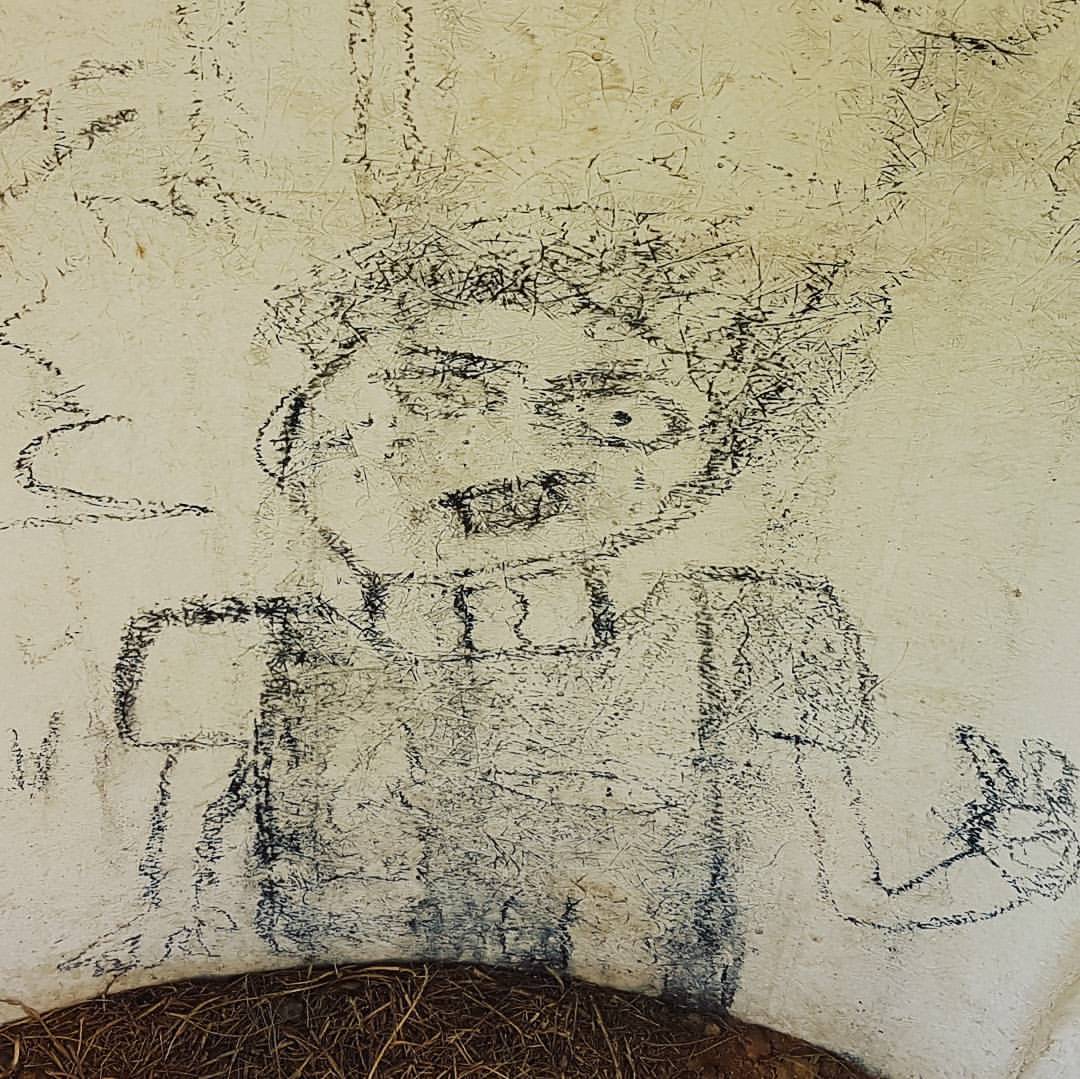A detailed sketch appears to be drawn directly onto a curved garden wall. At the base of the wall, there's a patch of dry, brown grass, enhancing the rustic and weathered aesthetic of the scene. The primary subject of the sketch is a haunting figure of a girl or woman, her face contorted in an expression of distress. Her hand is extended outward, and her hair is depicted as wild and untamed. The artist has masterfully integrated the wall's textured surface into the sketch, adding a layer of eeriness and depth to the artwork. The character's head is tilted at an unsettling angle, heightening the overall spooky and enigmatic feel of the piece.